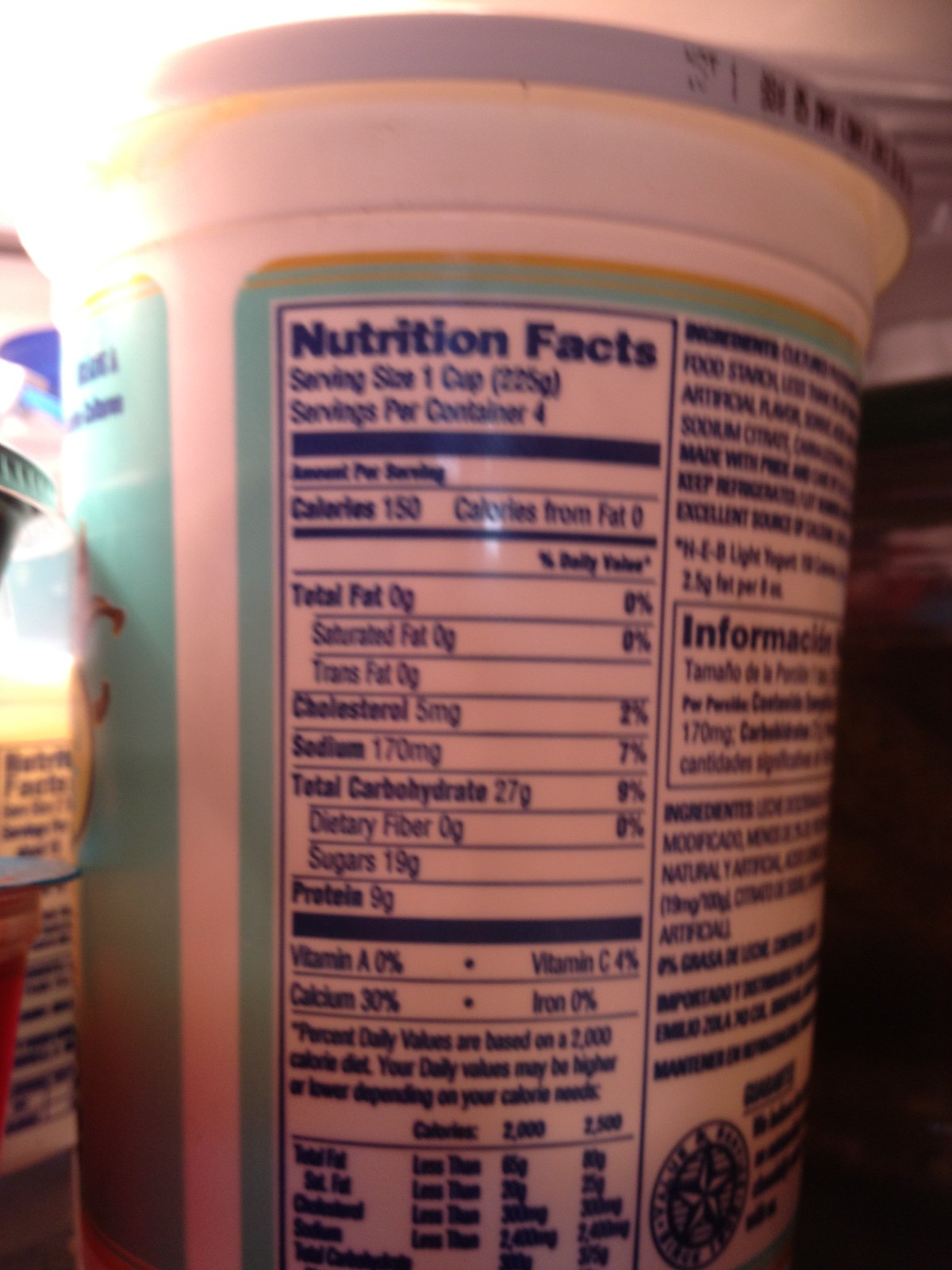The image showcases a white plastic container, possibly used for sour cream or yogurt, prominently featuring a blue-bordered nutrition facts label. The label details the serving size of 1 cup (225 grams), with 4 servings per container, and provides nutritional information such as 150 calories per serving, 0 grams of total fat, 5 milligrams of cholesterol, 170 milligrams of sodium, 27 grams of carbohydrates, of which 19 grams are sugars, and 9 grams of protein. It also notes the presence of 4% Vitamin C and 30% calcium based on a 2,000 calorie diet.

The container has a sea-green label with a gold trim around the top and a white lid marked with a sell-by date in black ink, which is partially obscured. Additional ingredients like food starch, artificial flavor, and sodium citrate are visible, though the container is angled, limiting full visibility of the list.

The setting appears to be inside a refrigerator, with light emanating from the fridge on the left side. Surrounding the main container are other items, including a bottle or container with its own nutrition facts label on the left and a red and white carton on the right, against a darker background.